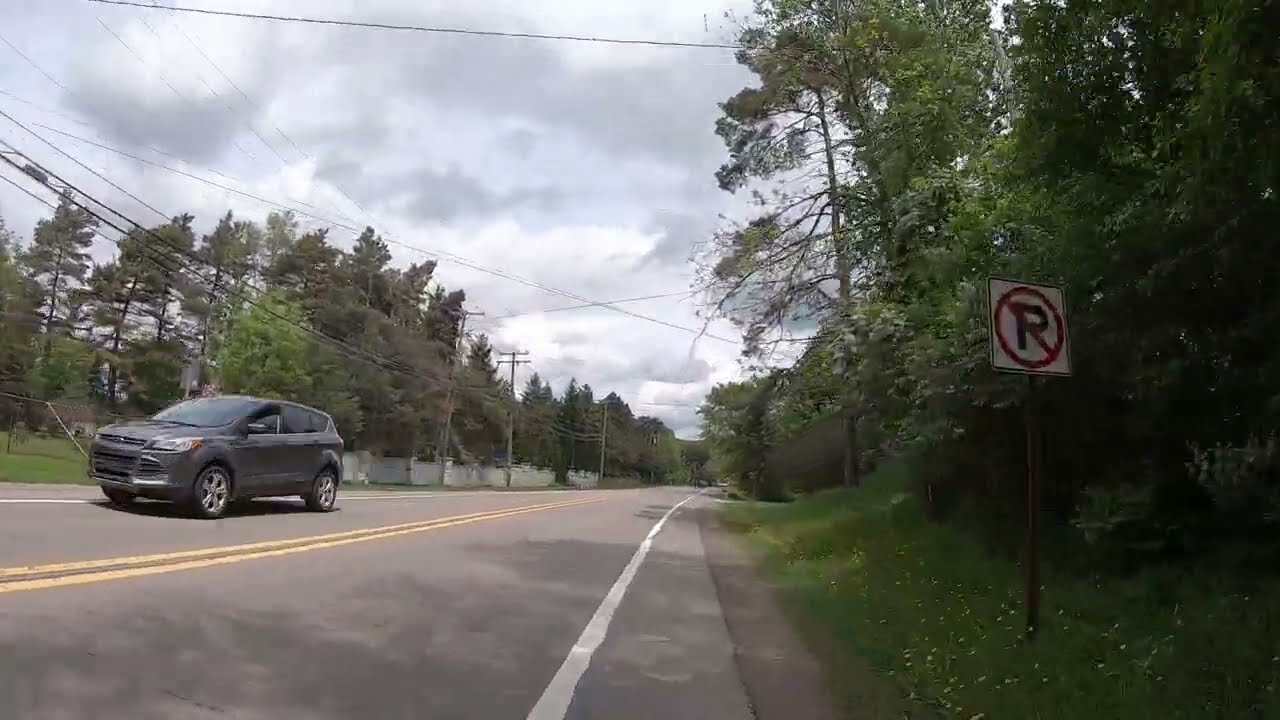The image depicts a cloudy day on a rural two-lane road divided by double yellow lines. A gray SUV, possibly a newer model minivan, is driving on the right-hand side of the road, heading toward the bottom left corner. Trees line both sides of the road, with a white fence running along the left side and a no parking sign oddly placed on the grassy verge to the right. Overhead, power lines cross from the left, though their poles on the right are not visible. There are patches of white flowers along the sides of the road, suggesting a spring or summer setting. Despite the natural surroundings, no buildings or houses are visible, making the presence of the no parking sign and scattered mailboxes seem out of place. In the far distance, another vehicle may be faintly visible. Overall, the scene is serene and somewhat enigmatic due to the juxtaposition of rural elements and suburban signage.